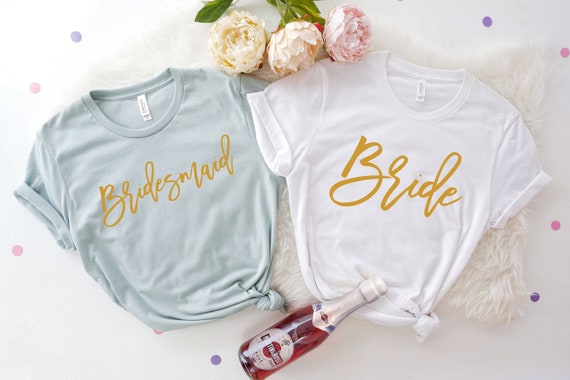This photograph provides a meticulously styled flat lay featuring two short-sleeved women's t-shirts and various decorative elements. The background is a white, thick, and slightly textured surface, likely a plush rug. A rectangular, white, hairy towel or small rug is positioned horizontally, serving as the base for the display and covering a significant portion of the frame.

On this soft surface lie two t-shirts, carefully arranged in parallel. To the left, there's a light green shirt with “Bridesmaid” scripted in a cursive, golden-yellow font across the chest. To the right, a white shirt bears the word “Bride” in a larger, matching font. Both t-shirts have their lower right corners tied into neat knots, adding a casual yet stylish touch to the scene. Each shirt also has a white tag visible at the back of the neck, emphasizing their new and unworn condition.

Further enhancing the composition is a small bottle resembling a champagne bottle, placed diagonally across the scene. The bottle's red liquid, reminiscent of cherry soda, contrasts vividly with the overall soft pastel tones. The bottle is slightly obscuring the “Bride” t-shirt, and it features a silver label at the top with a cork closure, adding a celebratory element to the layout.

Adding a touch of natural beauty, the tops of three flowers appear in the upper portion of the frame. The flowers, boasting full, fluffy petals, display a gradient of yellowish-white to vibrant pink colors, accompanied by a few green leaves, which create an elegant botanical accent.

Scattered across the white background surface are several small, pastel-colored circles in shades of pink and lavender, contributing a playful and festive atmosphere to the composition.

This highly detailed arrangement portrays a celebration theme, possibly hinting at pre-wedding festivities or bridal preparations, encapsulated in a cohesive, aesthetically pleasing visual narrative.